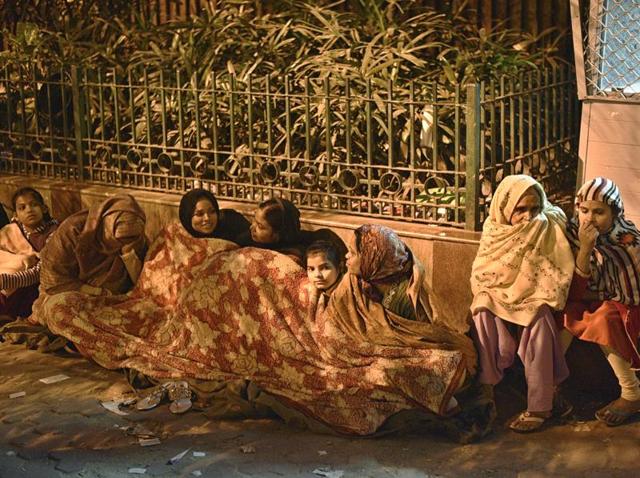In this photograph, a distressing scene unfolds, possibly in a war-torn or emergency-stricken area. The image captures a family huddled together on the ground, sheltered only by a carpet with reddish beige tones and gold designs, featuring turtles. This makeshift covering contrasts with their difficult reality. The family members, appearing desperate and uncertain, are partially concealed by the carpet, with their gazes wandering, searching for answers.

The backdrop consists of an iron fence set above a low wall, with plants visible behind it. Two women to the right, wearing hijabs and garments, are seen reacting to the harsh conditions; one covers her nose and the other covers her mouth with part of her hijab. In contrast, a person in the background stares at the family with a look of helplessness.

Given the attire of the people, this could potentially be in India or another region with similar traditional clothing. The overall atmosphere suggests homelessness and a dire need for shelter and relief amidst an apparent state of emergency. The poignant expressions and body language of the individuals encapsulate the hardship and uncertainty faced by those caught in distressing circumstances.